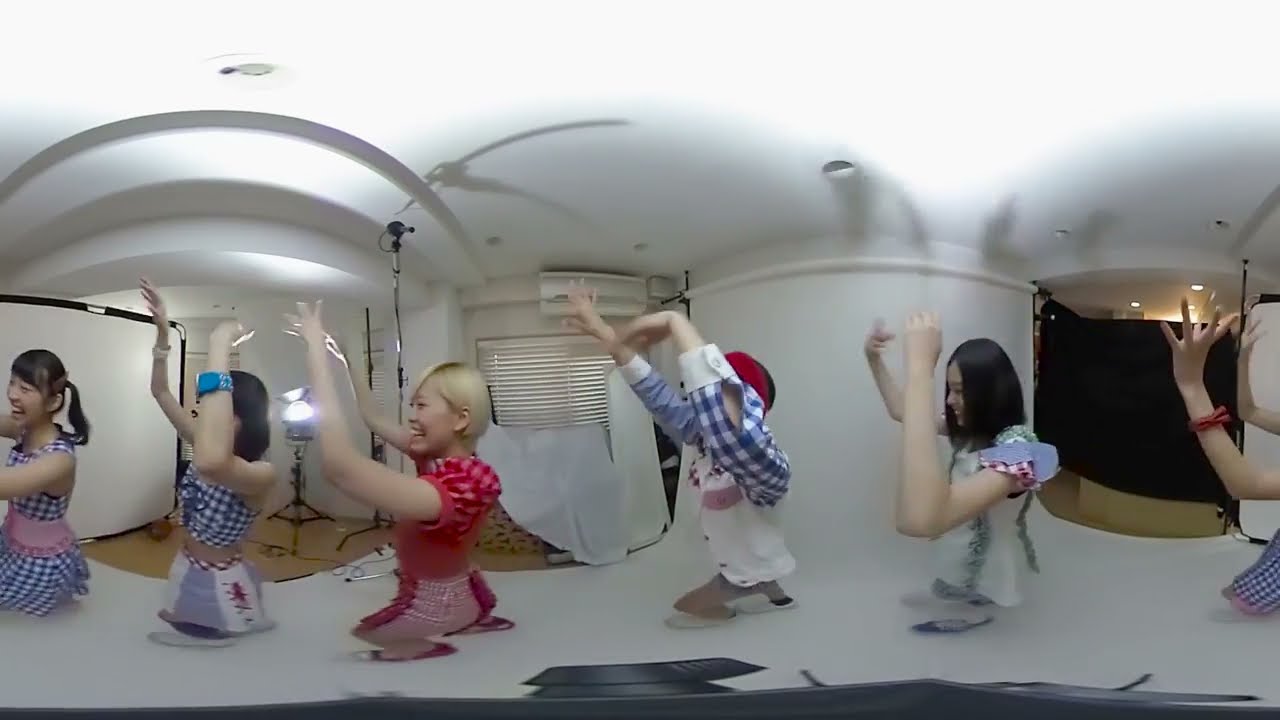This image captures a lively scene of several young Asian women, no older than their mid-twenties, engaged in a line dance within a predominantly white indoor room. The photo, taken with a fish-eye lens, adds a distinctive distorted perspective. The women, who stand one behind the other in synchronized positions, have their arms raised as if caught mid-dance. Most of the women have black hair, though one has short blonde hair. They wear coordinated outfits that blend modern and Western line dancing styles, featuring predominantly blue and white checkered patterns, with one woman sporting a red and white checkered outfit. 

The room itself is well-equipped with recessed ceiling lights, blinds on at least one window, a split AC unit on the wall, and a screen. A stage light and a large whiteboard are positioned to the right, next to a blackout curtain and a white tarp covering most of the beige floor. The setup suggests a space prepared for filming or a television program, enhancing the dynamic and energetic atmosphere of the dancers.